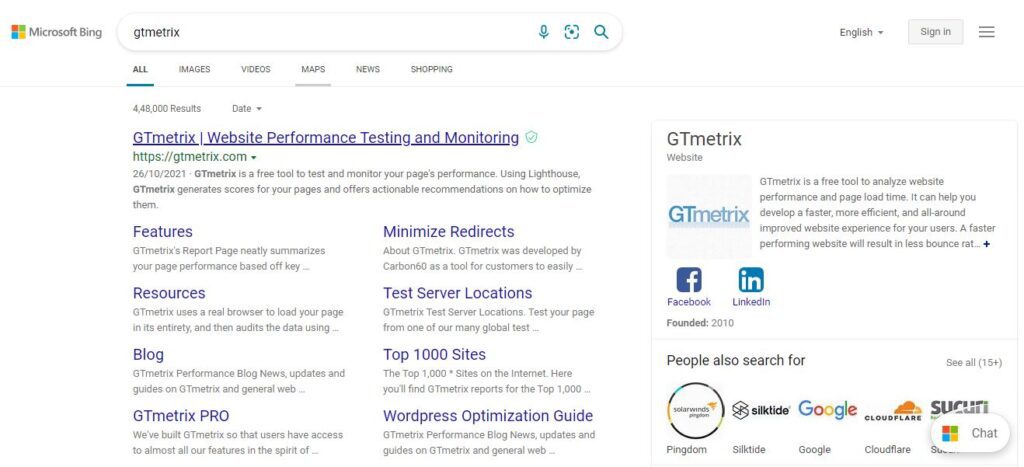Screen capture of a Microsoft Bing search results page with a white background. In the upper left corner, the iconic Microsoft logo is displayed, consisting of four squares in red, blue, yellow, and green. To the right of the logo, the text "Microsoft Bing" is clearly visible. Adjacent to this, a search box contains the typed query "GTmetrix."

Below the search box, a navigation menu with search options is shown, delineated with underlined text. The options "All," "Images," "Videos," and "Maps" are underlined in blue, whereas "News" and "Shopping" are underlined in gray, indicating the default selection.

The main portion of the screen displays the search results. The top result is a clickable link with the text "GTmetrix / Website Performance Testing and Monitoring," underlined to signify a hyperlink. Directly beneath the hyperlink, the web address "https://GTmetrix.com" is written in green text, confirming the official webpage for GTmetrix.